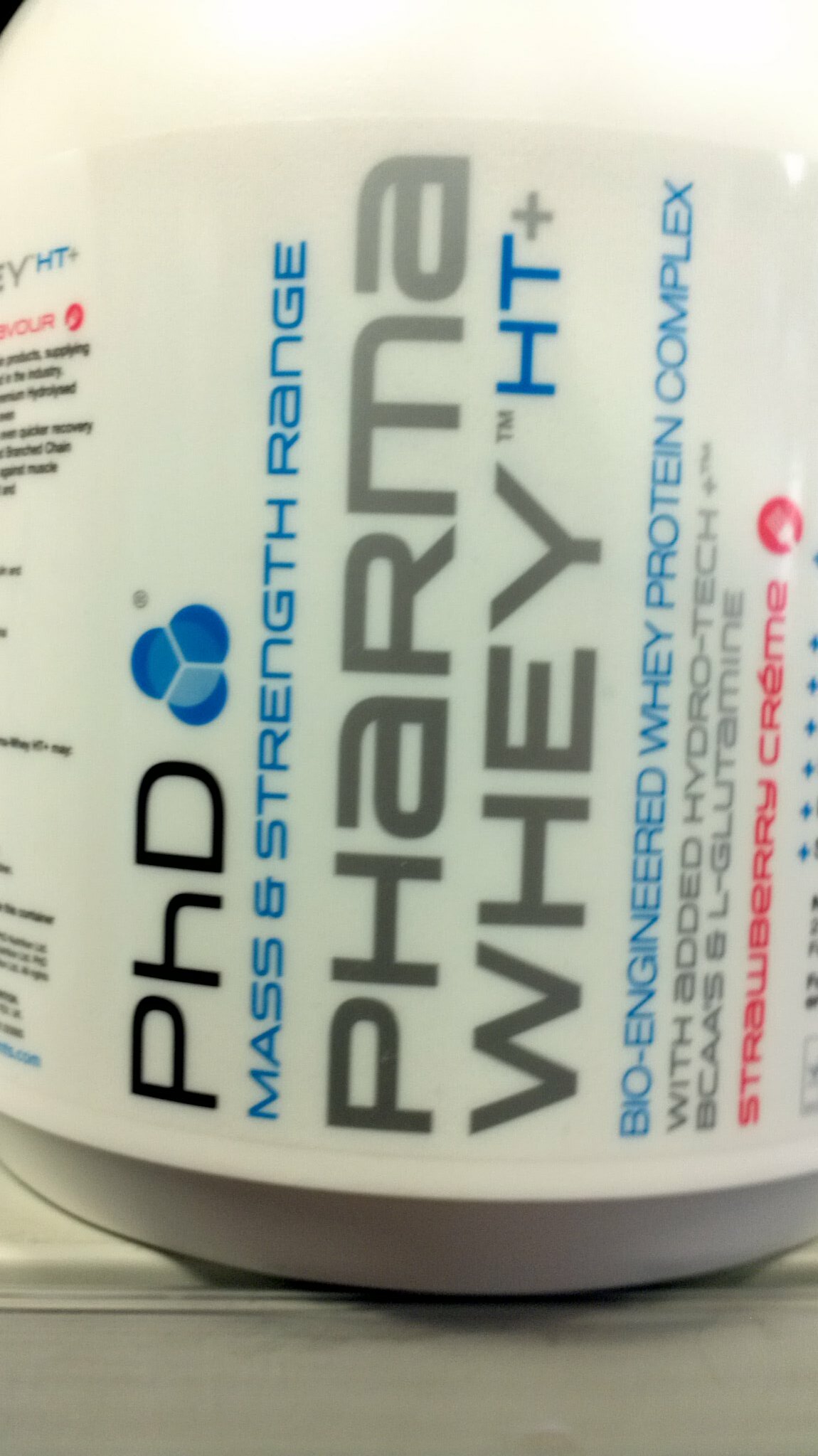The image features a large cylindrical container, likely made of metal, with a silver bottom. The container, possibly a can or jar, has a closely cropped composition leaving no external context or scale reference. A white or transparent label with white granular contents visible through it covers the container. Prominently displayed on the label are the large black letters "PhD," accompanied by a blue floral-like design formed by three semicircles overlapping. Below this, the label reads "Mass and Strength Range" in blue. Further down, the text "Pharma Whey HT+" is printed, with "Pharma Whey" in gray and "HT+" in blue. At the bottom of the label, "Bioengineered Whey Protein Complex" is inscribed in blue. Extra details in red, blue, and black are situated at the far left and right edges of the label, though their specifics are not entirely clear.